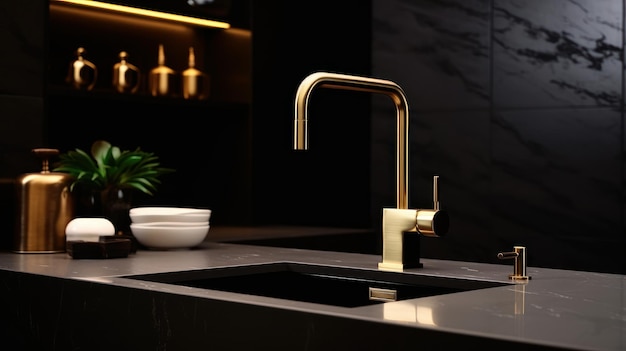This photograph captures a sleek, modern kitchen featuring a focal point of a chic sink and faucet arrangement. The countertop, crafted from dark gray material, supports a large, square, single basin sink and an ultra-modern faucet that combines brushed and polished gold finishes. There's a single stark handle attached to the faucet, exuding minimalist elegance. Located beside the sink is a small collection of white bowls and a lush green leafy plant, adding a touch of natural vibrancy. Also present is a gold soap dispenser and what appears to be a gold ice holder. Above the scene, four gold-tinged glasses hang from a shelf. The background is a stylish black wall, gradually transitioning to a brighter hue towards the right, with distinctive hanging Edison bulbs on a track system subtly out of focus to the left. The entire setting is professionally illuminated, spotlighting the sink and its surroundings, while the bottom of the image fades into a darker shade, contributing to the room's sophisticated atmosphere.